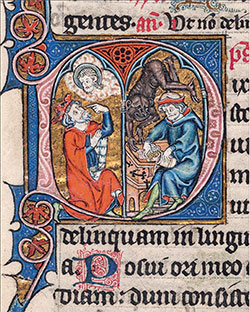The image, likely an excerpt from a book or newspaper, with a light gray background, features ornate calligraphy text in a foreign language. These texts, primarily black with some words in red or blue, are written with calligraphy pens. The left side of the picture showcases a man in a blue suit and red cape, wearing a crown and looking upward towards an angelic figure in the sky. This character also has a red band around their head. To the right, another figure in a blue robe with a hood, also adorned with a red band, looks downward, while behind him, an upside-down demon menacingly looms. The image is detailed with additional design elements along the border in blue and red and features major colors including red, blue, black, and shades of brown.